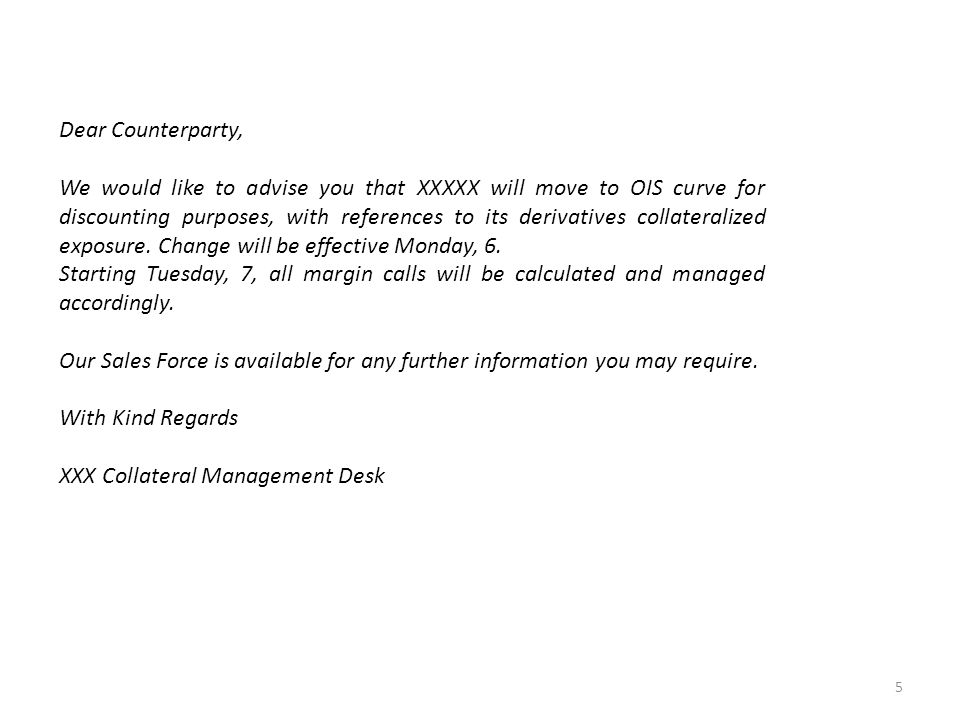The image portrays a letter or email written in black skinny text on a completely white backdrop. The letter begins with "Dear Counterparty," and proceeds to advise that XXXXX will move to an OIS curve for discounting purposes, referencing its derivatives and collateralized exposure. The document specifies that the change will be effective starting Monday, the 6th. Following this, it indicates that from Tuesday, the 7th, all margin calls will be calculated and managed accordingly. A subsequent paragraph assures that "our sales force is available for any further information you may require." The letter concludes with "With kind regards," followed by "XXXX Collateral Management Desk" at the center of the page.